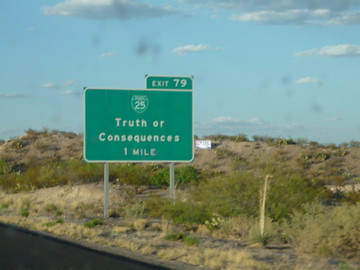Under the expansive blue sky scattered with fluffy white clouds, the arid landscape features a mix of sun-bleached yellow grass and sporadic patches of resilient green. Sturdy metal posts anchored in the dry earth support a green highway sign indicating "Truth or Consequences - 1 Mile" alongside a notice for "Exit 79". To the left of the scene, a stark black asphalt road slices through the predominantly dry desert area, epitomizing the rugged, open terrain that stretches into the distance.